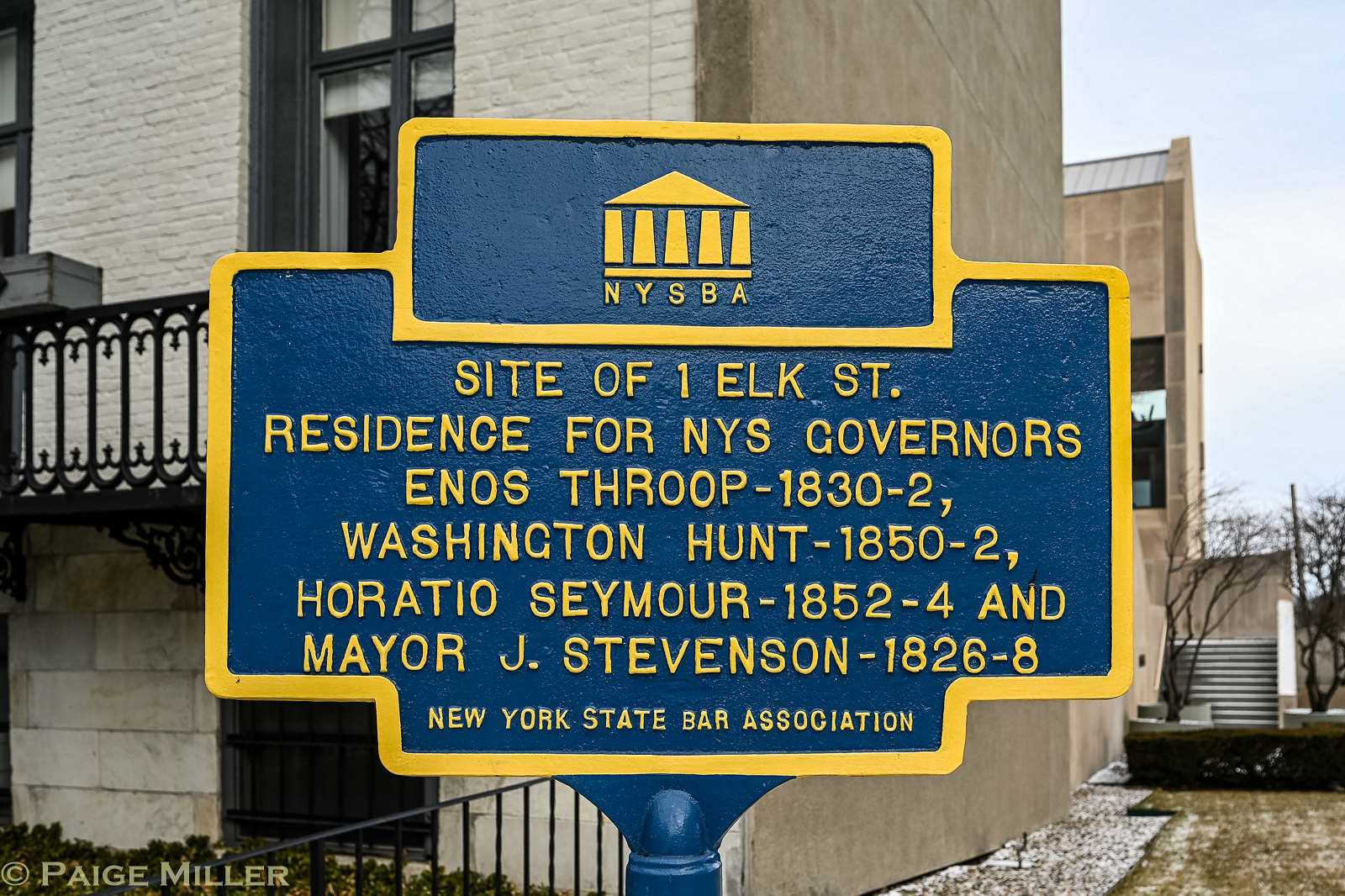This image is a close-up of a prominently displayed sign on a post, situated outdoors with a backdrop of buildings featuring white-painted bricks, windows, and a metal walkway fence. The sign has a distinct medium blue background with gold trim and lettering. At its top, the sign features the emblem of the New York State Bar Association, depicted as a gold triangle roof supported by five pillars. Below the emblem, the letters "NYSBA" are prominently displayed. The inscription that follows reads: "Site of 1 Elk Street, residence for NYS Governors Enos Throop 1830-1832, Washington Hunt 1850-1852, Horatio Seymour 1852-1854, and Mayor Jay Stevenson 1826-1828." At the bottom, the sign bears the name "New York State Bar Association." The setting is enhanced by the presence of adjacent buildings, including an apartment building with balconies and stairs, contributing to the urban atmosphere of the scene.